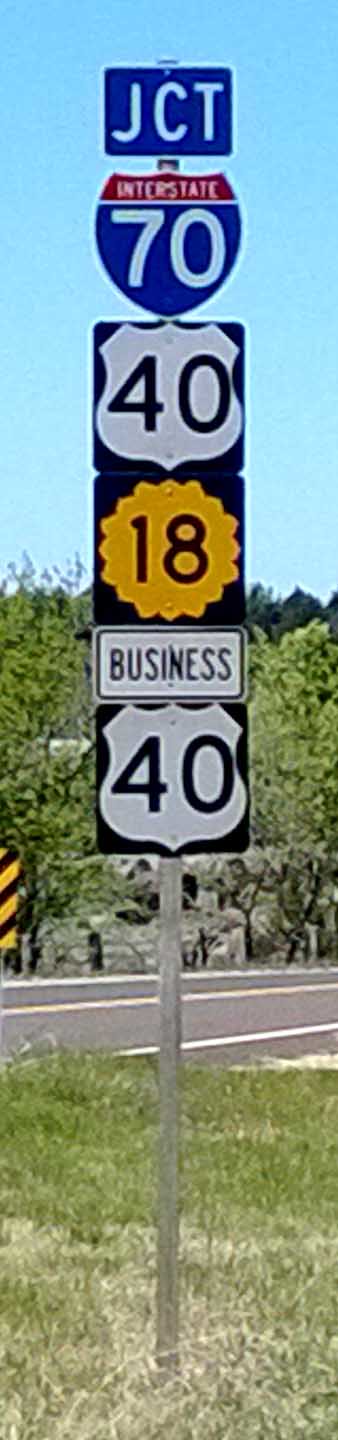The tall, narrow image captures a section of a two-lane highway bordered by rugged rocks, likely cut through to make way for the road. Dominating the upper portion of the image is a bright blue, cloudless sky, with a backdrop of trees and dense vegetation. Towards the middle, the top of the trees can be seen lining the rock ledge, descending to meet the highway that stretches from left to right. In the foreground, a patch of grass, greener and fuller away from the base but dryer nearby, frames a metal pole adorned with multiple traffic signs. At the pole's pinnacle is a blue sign with white lettering indicating 'JCT' for junction, followed by a shield-shaped red, white, and blue interstate sign for Interstate 70. Beneath it, a black sign with a white shield design indicates US Highway 40. Further down is a distinctive yellow sign with wavy edges displaying the number 18. Another sign below points to 'Business 40'. Additionally, there is a duplicate sign for US Highway 40. On the far left side of the image, across the road from the viewer, a diagonally striped black and yellow warning sign stands out.